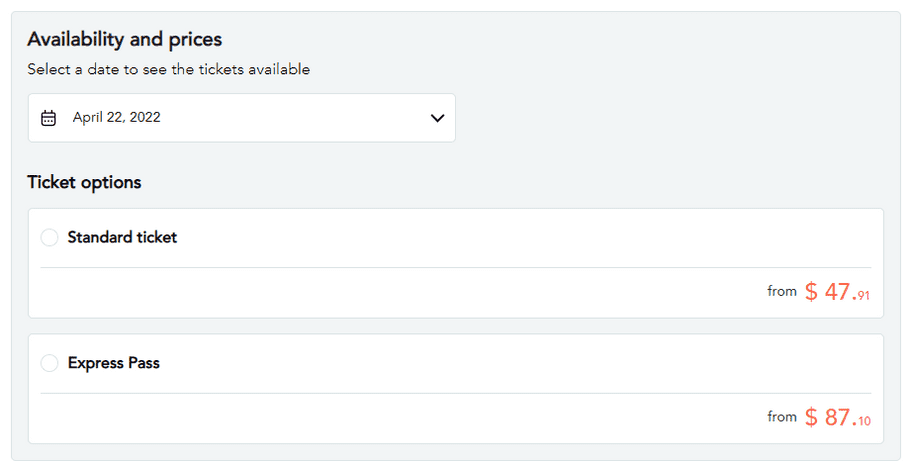This image is a screenshot of a menu from a website displaying ticket availability and pricing options. The background is light gray, and the content is aligned to the upper left corner. The heading "Availability and Prices" is prominently displayed in bold black font. Below this heading, a smaller black font instructs users to "Select a date to see the tickets available."

A white drop-down field titled "April 22, 2022" is situated below this instruction, featuring a calendar icon on the left and a downward-pointing arrow on the right, indicating its drop-down functionality.

Further down, the section titled "Ticket Options" appears in bold black font. Within this section are two choices:

1. **Standard Ticket**: Displayed inside a white rectangle, this option includes a selection circle next to the bold text "Standard Ticket." In the lower right corner of this rectangle, it indicates the starting price with the text, "From $47.91."

2. **Express Pass**: Similarly, this option is enclosed within a white rectangle featuring a selection circle. Next to it, the bold text reads "Express Pass," with the lower right corner highlighting the starting price "From $87.10."

Overall, the menu is a straightforward and user-friendly pop-up designed for selecting ticket options on a specific date.